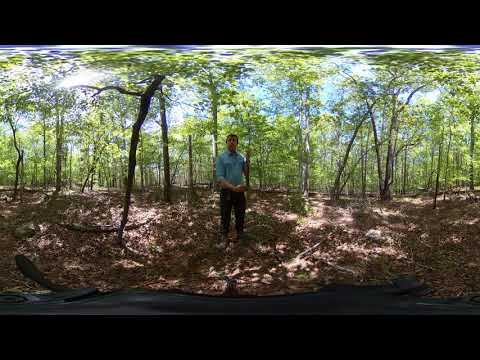The image depicts a Caucasian man with light brown hair standing in a wooded area on a ground covered in brown leaves and some branches. He is wearing dark blue pants and a light blue collared shirt with sleeves that extend just below his elbows. He is holding up a long object with his right hand and pointing at it with his left hand; while the exact nature of the object is unclear, it resembles a stick or possibly a firearm. The wooded area around him is dense with very thin, small trees adorned with vibrant green leaves. The background features a blue sky with white clouds, and sunlight filters through the leaves, casting a reflective glow. The image has a slightly distorted appearance, possibly indicating it was taken in panoramic mode. There are black strips across the top and bottom of the image, adding a framed effect to the photograph.